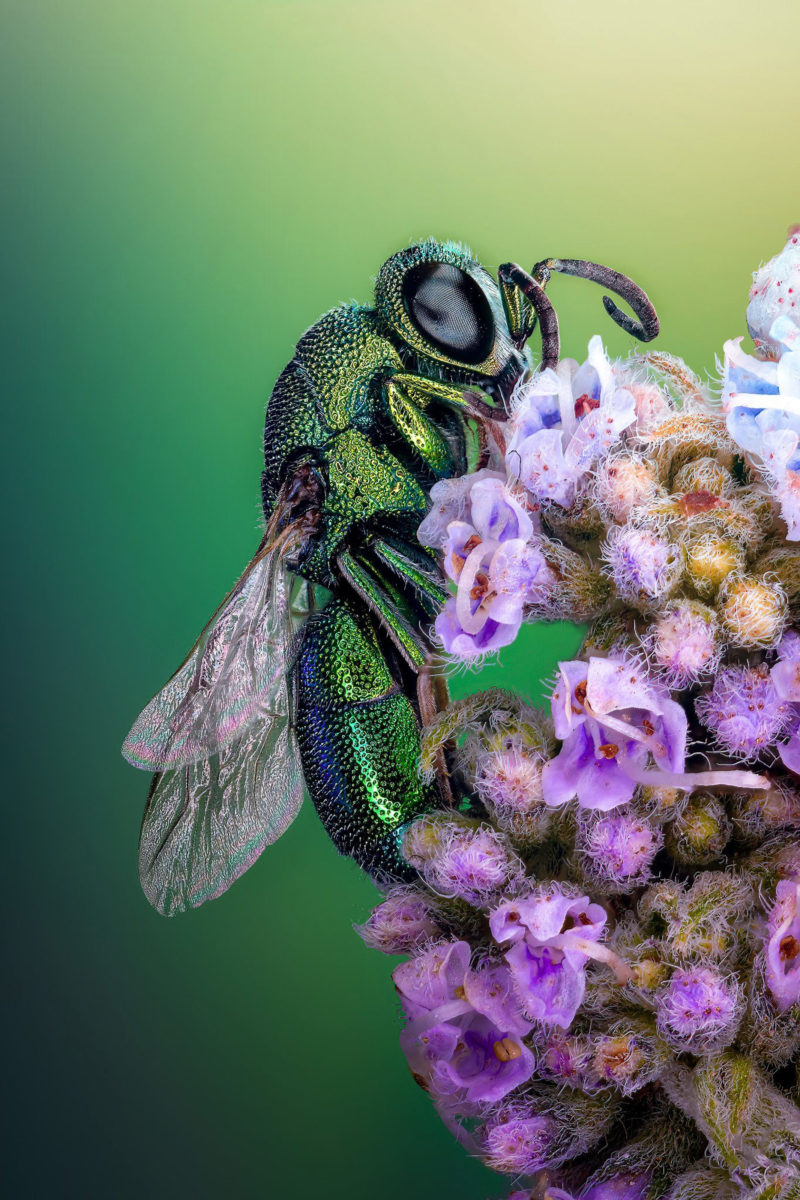This high-resolution digital artwork features an extremely lifelike yet otherworldly depiction of a fly. The image is oriented in a portrait format, showcasing a close-up, side profile of the fly, from its vertical head at the top to its tail end at the bottom. The fly’s body exhibits a stunning iridescence, transitioning between deep green and blue hues depending on the light. Its head is dominated by a large, almost entirely black eye, with two small, curly antennae extending outward. The thorax is adorned with relatively short, translucent wings that shimmer in the light. The abdomen is slightly larger than the thorax, adding to the insect's alien-like appearance.

The fly is perched on a vibrant cluster of purple flowers, some of which are fully bloomed while others remain in bud form. The background enhances the surreal quality of the image, featuring a gradient of various shades of green that transition from dark at the bottom to light at the top. The overall green backdrop provides a striking contrast to the purple flowers, drawing the eye to the intricately detailed fly, which appears almost too fantastical to be real. This visually captivating image, with its fluorescent colors and reflective hues, combines elements of both nature and imaginative artistry, creating a vivid and mesmerizing scene.